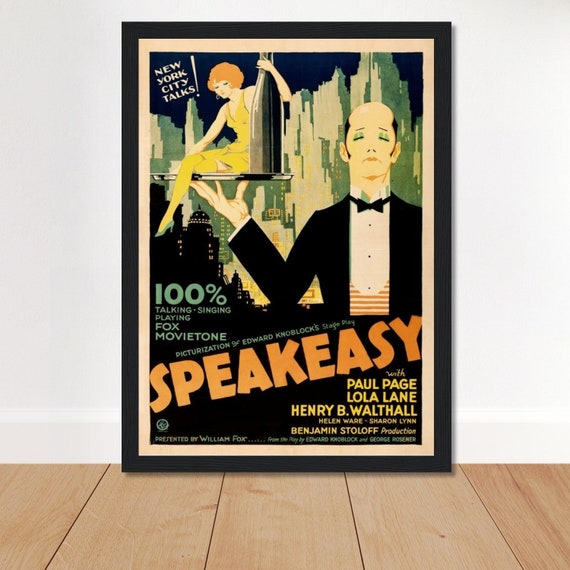The framed poster, leaning against a pastel blue wall on light tan hardwood flooring, features a vintage 1940s-style illustration advertising "New York City Talks." Dominating the upper left corner, the title is accented with a long, skinny white exclamation point. A central cartoon image depicts a tuxedo-clad waiter holding a tray on which a woman with curly red hair, adorned in yellow stockings, a yellow dress, and earrings, perches. Her right leg dangles over her left, completing her ensemble with a blue shoe. She is posed with her arm around what appears to be half of a wine bottle. Surrounding this scene is a backdrop of New York City. The poster promotes 100% talking, singing, and playing by Fox Movietone, highlighting the picturization by Edward Knobloch of his stage play, "Speakeasy," with credited stars including Paul Page, Lola Lane, Henry B. Walthall, Helen Ware, Sharon Lynn, and Benjamin Stoloff. The artwork is bordered by a white margin, framed in black, and situated against the hardwood floor with five and a half panels visible.